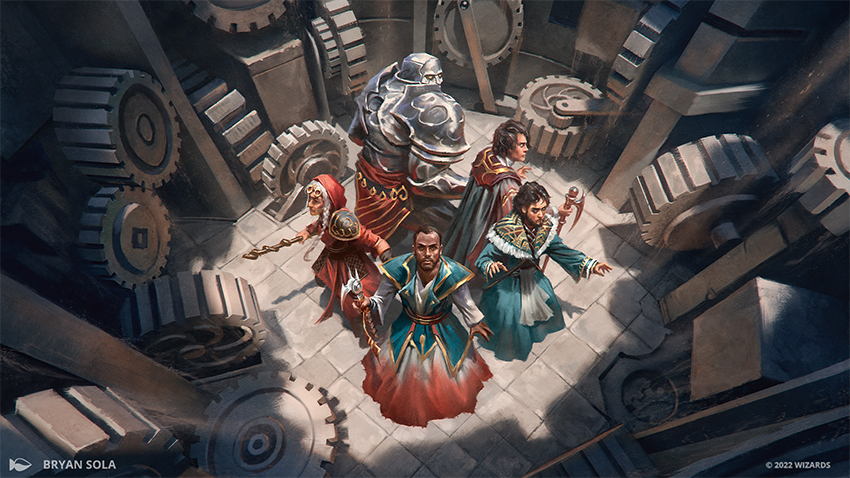The image depicts a scene that appears to be from a video game, showcasing a group of five characters, whose attire blends traditional wizard outfits with modern and fantasy elements. They are positioned in the center of the image, surrounded by heavy machinery such as large metal gears and circular knobs, giving an industrial atmosphere. The characters are diverse in appearance; some don turquoise and red mage robes, while others wear warrior-style armor, with one character even resembling a robot clad in metallic gear. They all brandish weapons and stand on a tiled floor, radiating a sense of readiness for combat. The bottom left corner of the image features the name "Brian Sola," presumably the creator, while the bottom text reads "2022 Wizards," suggesting a possible title or theme related to the depicted scene.